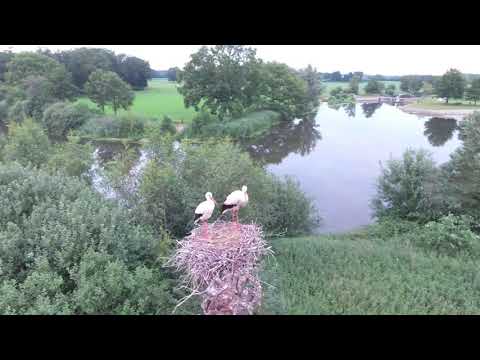In the foreground of this nature scene, two long-legged waterfowl, resembling a mix between seagulls and herons, are perched on a large nest made of twigs and branches. The birds are predominantly white with black-tipped wing feathers. The nest is situated at the edge of a tranquil pond or small lake, bordered by tall brush and bushes. The water behind the nest reflects the light, creating areas of varying brightness. Surrounding the water, the background is rich with green trees and shrubbery, with patches of grass visible in the upper corners of the image. There also appears to be a flat, open area along the lake's perimeter, which might serve as a beach or a boat launch.